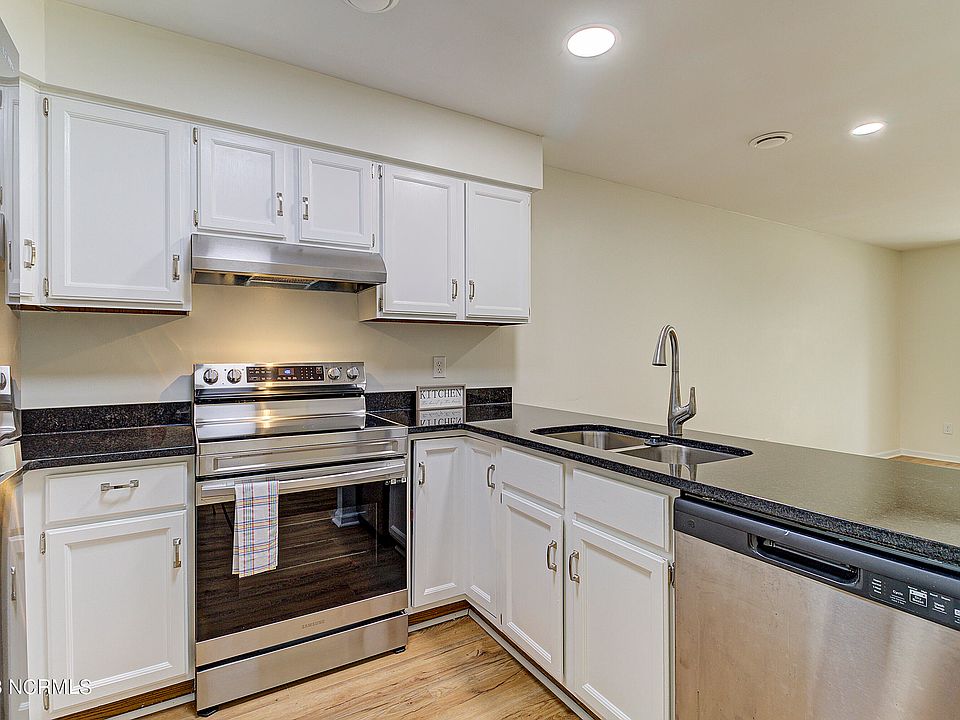This photograph captures the interior of a vacant, modern L-shaped kitchen, likely part of an apartment. The kitchen features sleek black marble countertops, including a peninsula that faces an adjoining empty room, which could serve as a dining or living area. Prominently displayed on one of the counters is a sign that says "kitchen." 

The appliances are chrome, with notable items including a silver dishwasher positioned next to a double sink. Above and below the countertops are white cabinets with stainless steel handles, providing ample storage space. The oven and stove are located along the farthest back wall, accompanied by a range hood for ventilation. The kitchen is illuminated by several ceiling lights, highlighting the refined finish of the countertops and cabinets. No furnishings are present in the adjoining room, emphasizing the vacant nature of the home.